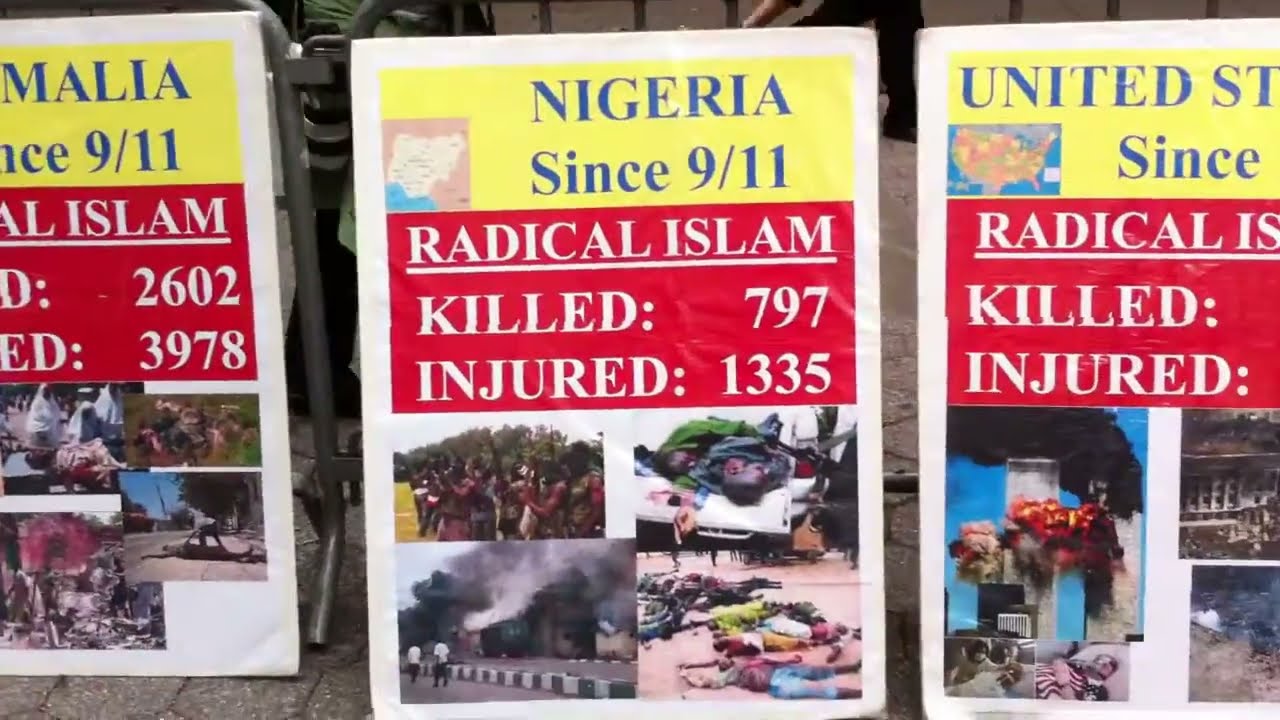The image depicts three large posters placed in front of metal railings, suggesting a protest or public demonstration. Each poster focuses on the impact of Radical Islam since 9/11. 

The left poster appears partially visible, featuring a title related to Malia. It includes numbers "2602" and "3978" in white text against a yellow backdrop, surrounded by various images. 

The center poster is fully visible and more detailed. It displays "Nigeria" in blue text above a subtitle "since 9-11." Below, a red rectangle contains the text "Radical Islam killed 797 injured 1335," also adorned with images of victims and casualties, along with a small map of Nigeria in the bottom left corner.

The rightmost poster also uses blue text, partially reading "United ST" followed by "since 2011." It lists casualties with the text "Radical Islam killed and injured," against a red background. Images of the 9/11 attacks and other destructive scenes fill the remaining space. 

All three posters have white borders and are propped up on the ground, possibly against a wall or fence, with paving stones beneath and onlookers standing behind the barriers. The overall setup conveys a strong visual and textual narrative on the casualties attributed to Radical Islam in different regions since 9/11.